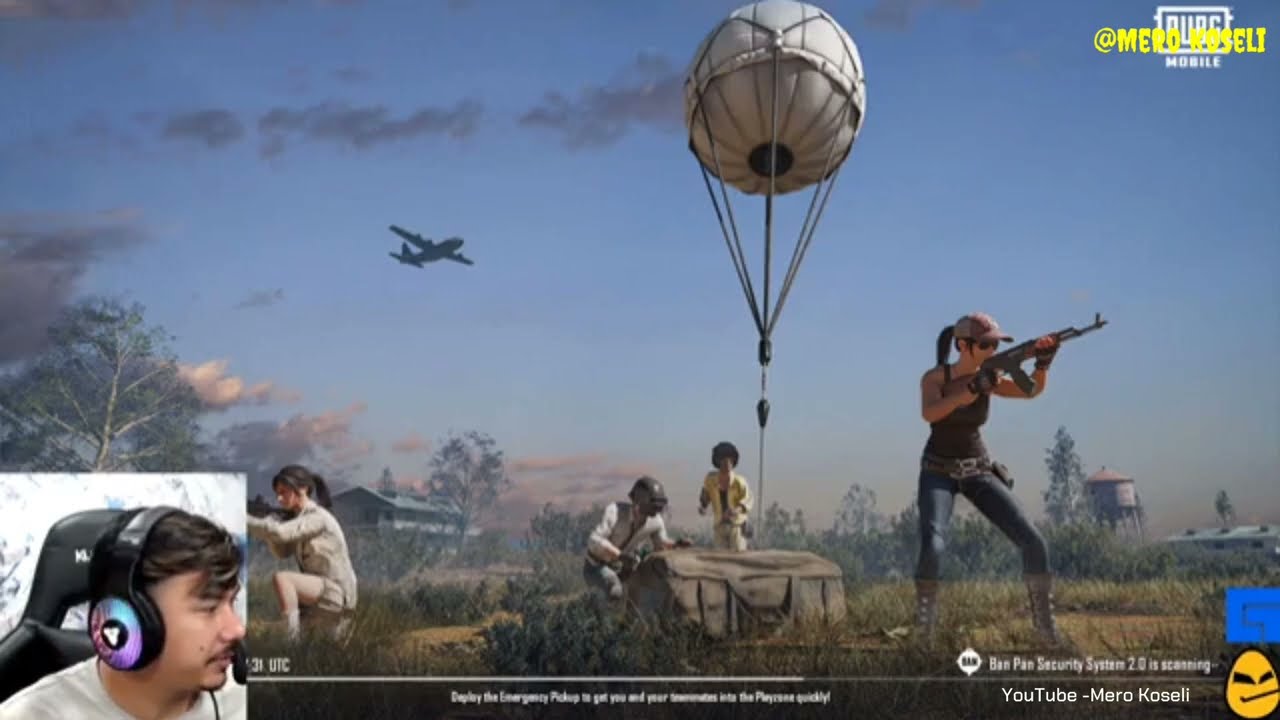The image is a detailed screenshot from a live stream of the game PUBG Mobile. In the upper right-hand corner, the text "@morrowcoseli" is displayed in yellow, partially obscuring "PUBG Mobile." In the bottom right-hand corner, it reads "YouTube Morrow Coseli." In the lower left-hand corner, there is a small window showing the streamer, a light-skinned man with brown hair, wearing black LED-illuminated headphones, seated in a black gaming chair.

The gameplay scene is in 3D, featuring a vibrant blue sky with an airplane flying overhead. A white air balloon is tethered to a rectangular loot crate, draped with a tan blanket. The scene includes multiple characters: two women armed with AR-15-style guns, one standing and the other kneeling, seemingly guarding the crate. Two additional figures, whose genders are not clearly identifiable, are running toward the loot crate that appears to have just been dropped from the sky. The background showcases a house, numerous trees, a water tower, and an overall lively environment indicative of cooperative gameplay.